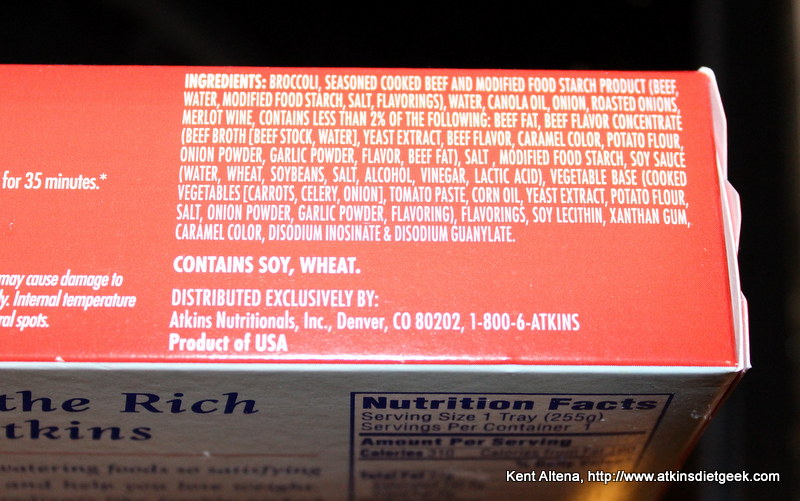This image showcases two distinct sections of a product box. The upper section features the top side of the box, detailed in a light red background adorned with white text on the left. Here, a paragraph outlines the ingredients list, followed by additional information stating the presence of soy and wheat, and the distributor's details. The lower section of the image captures the back side of the box, revealing the upper half of the nutrition facts label set against a gray background. Notable on the bottom right corner of the image, in small white lettering, is the text "Kent Altena, http://www.atkinsdietgeek.com." A consistent black background frames the image on the top and right sides.